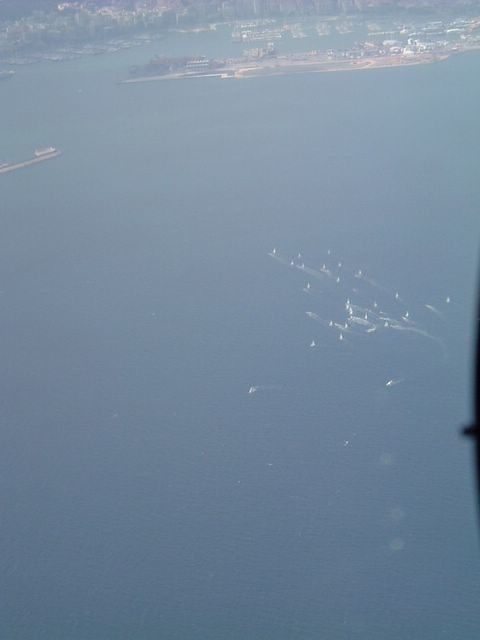The aerial photograph, likely captured from a helicopter or drone, provides an expansive view of a large body of water, possibly a bay or wide river estuary. Dominating the foreground is this dark turquoise-blue water, dotted with numerous small white shapes, possibly fast-moving sailboats leaving subtle wakes, giving the impression of a boat race. A thin, black sliver marks the very edge of the image, hinting at an unspecified object just out of frame. In the upper portion of the photograph, a somewhat hazy and washed-out landmass can be seen, featuring brown and green tones, indicating grassy and tree-covered areas. This landmass includes a small peninsula with what appears to be docks or a marina, where boats are uniformly parked in rectangular formations. Behind the peninsula, the blurred outlines of a town or city are faintly visible, with gray and brown buildings standing against the horizon. The overall scene is slightly blurry and pale, suggesting it might have been taken on a hazy day, but the intricate details, such as the scattered boats and the structured marina, provide a captivating and descriptive snapshot of this coastal region.